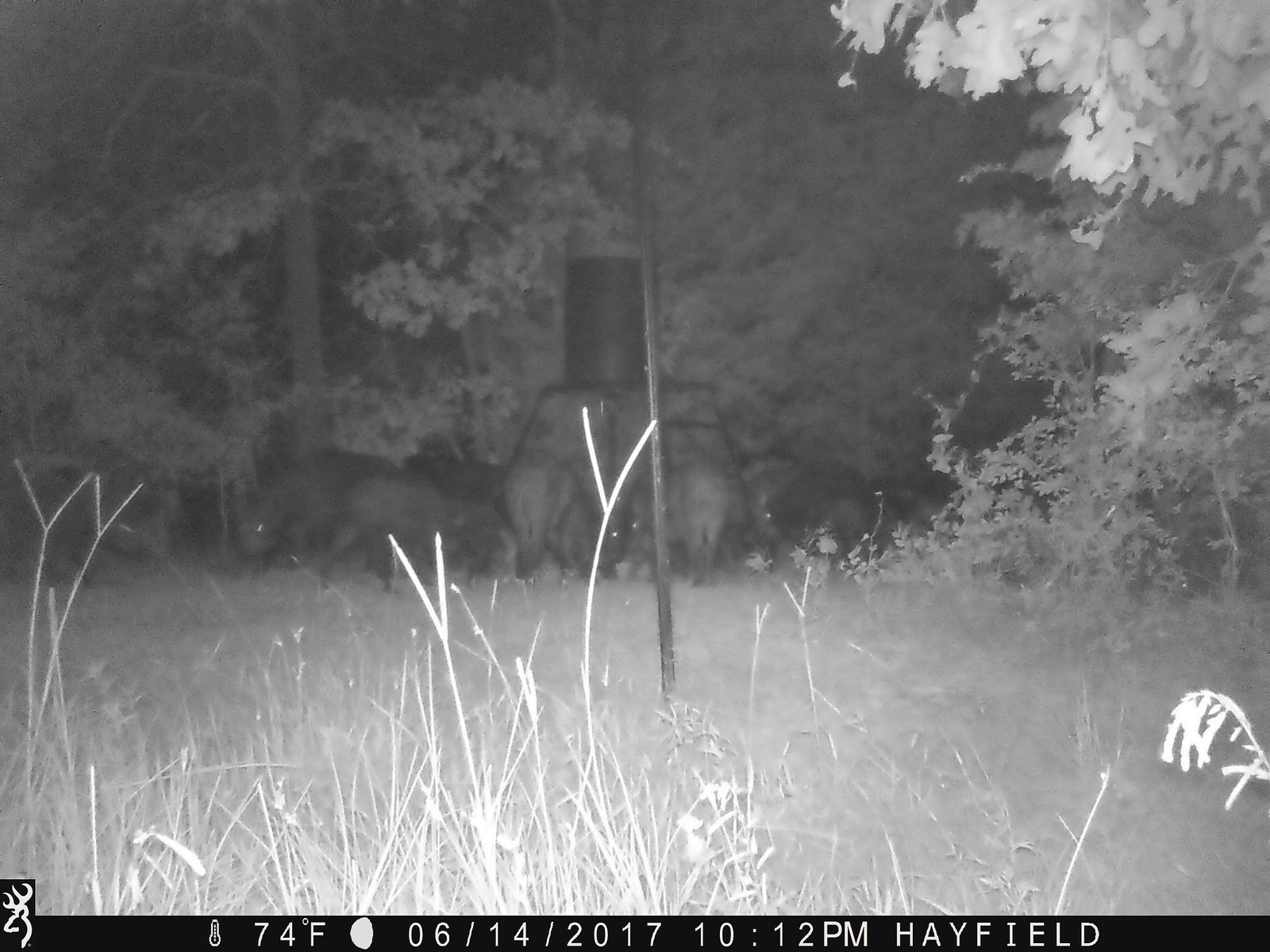This black and white photograph, taken on June 14th, 2017 at 10:12 p.m. with a temperature reading of 74 degrees Fahrenheit, captures a blurry nighttime scene possibly intended for hunting or wildlife observation. The image seems to be from a night vision or game camera, indicated by the reflective, glowing eyes of several indistinct animals in the middleground, partially obscured by thin grass and brush in the foreground. The distant background shows a cluster of trees, with some highlighted areas in the top right. A metal pole stands prominently in the middle, supporting a cylindrical metal object, potentially a bird feeder. The bottom border of the image includes icons such as a deer with antlers, a temperature gauge, and a moon phase indicator, alongside text specifying the location as "Hayfield" and the exact time and date.